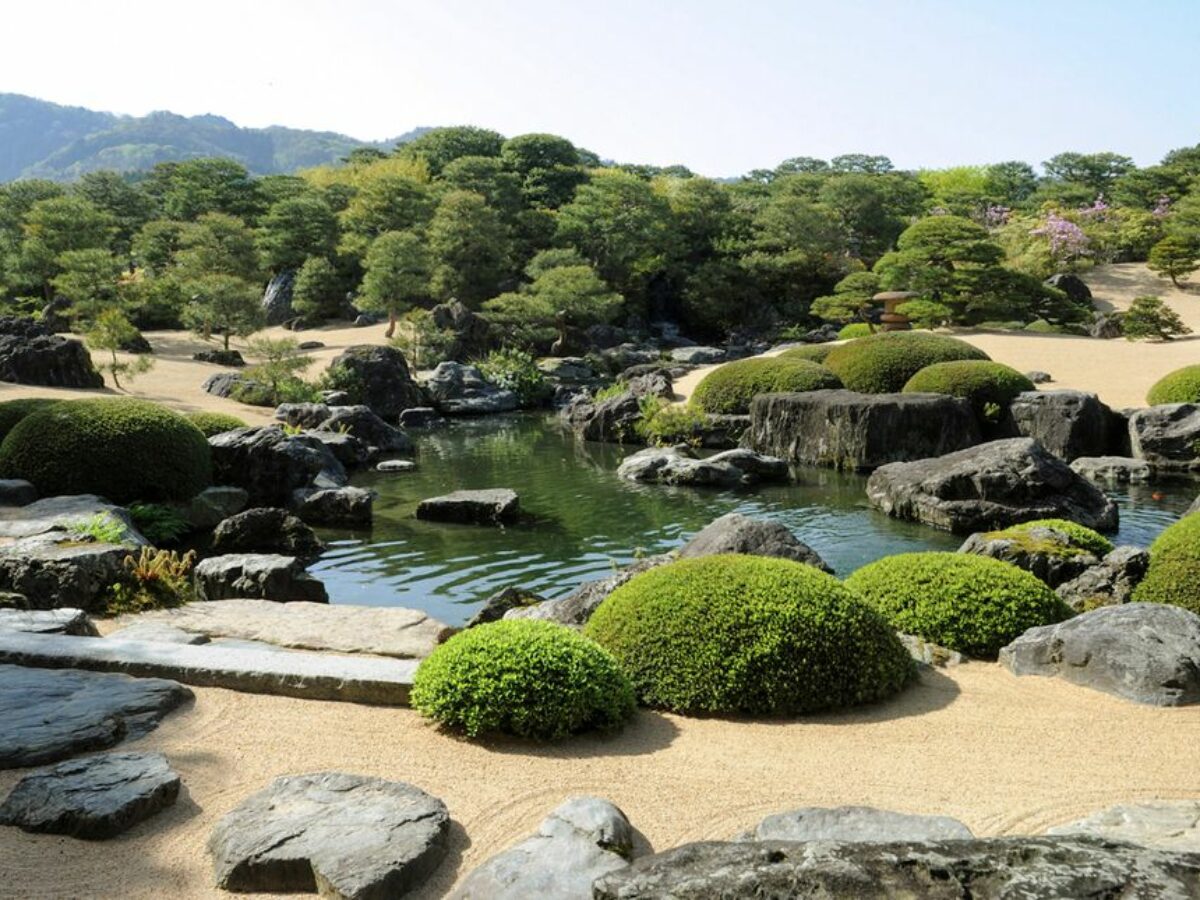The image depicts a serene natural outdoor environment, likely a park, as viewed from a slightly elevated vantage point. At the bottom, large gray rocks rest on a sandy surface, interspersed with perfectly symmetrical, circular green hedges. Gradually moving upwards, these hedges border a tranquil, man-made pond with greenish water, featuring smooth-topped rocks that both protrude from the water and frame its edges. To the left, steps lead down to the pond, suggesting careful landscaping.

Further into the background, the sandy or possibly grassy terrain slopes gently upwards, eventually giving way to a dense forest of trees. These trees vary in shape but include distinctive dome-like tops similar to the meticulously pruned hedges near the pond. Adding a splash of color, pinkish flowers can be seen on the left side of the image. Above all, the backdrop transitions into a sky of light blue and gray hues, evoking a calm and peaceful atmosphere.